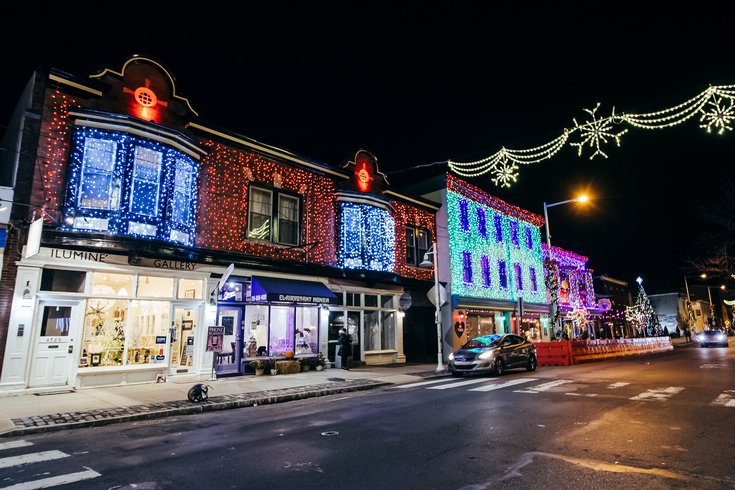This detailed, unified caption transforms the provided inputs into a single descriptive account:

---

This image captures a picturesque vintage downtown area beautifully decorated for Christmas at nighttime. The scene features charming, antique two-story buildings, each extensively adorned with colorful holiday lights. The building on the left prominently displays the sign "ILLUMINE Gallery," with its facade embellished in festive red and blue lights. The second story of this building is particularly radiant, covered entirely with sparkling red and blue lights. Adjacent to it, slightly out of focus, is a building with an awning and vibrant red and blue lights, although the text on the awning is not fully clear. Further to the right, another building stands out with its windows glowing in deep blue, while its front sparkles with green lights. The rooftops of the buildings are accented with darker red lights, enhancing the overall festive atmosphere.

Crossing the paved, slightly wet street, suspended Christmas lights and snowflake decorations create an enchanting canopy above, adding to the magical Christmas scene. The sky is pitch black, making the colorful lights and the gently glowing streetlights stand out even more. A single car is parked on the street, contributing to the quiet, serene feel of this night. Crosswalks lead up to the various businesses, inviting passersby to enjoy the festive and inviting retail area.